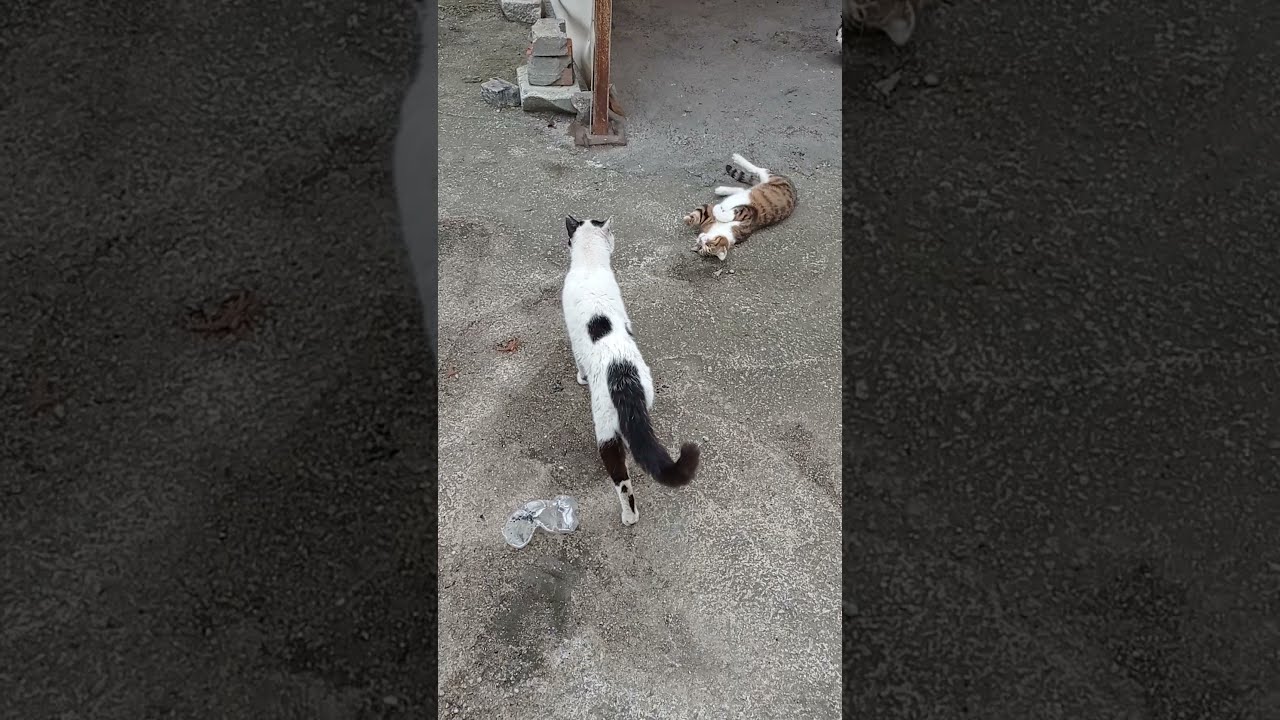The image is a vertical cell phone photo of two cats on a unique, grayish, thick sand or gravel surface in an outdoor setting. The photo is presented in a rectangular format with darkened panels on either side, highlighting the central image. In the foreground, walking away from the camera, is a predominantly white cat with distinct black markings on its head, including a van pattern of two black spots, and a black tail. Beside this cat, there is a piece of broken plastic bottle. Additionally, in the background to the right, there is a second cat lying on its back with its paws extended upward. This cat has a white belly and white paws, with an orange and black tabby pattern. Surrounding the cats, the scene includes pieces of concrete, a rusted fence post, a white fence, a stack of bricks, and some scattered rocks, providing a detailed and textured backdrop.